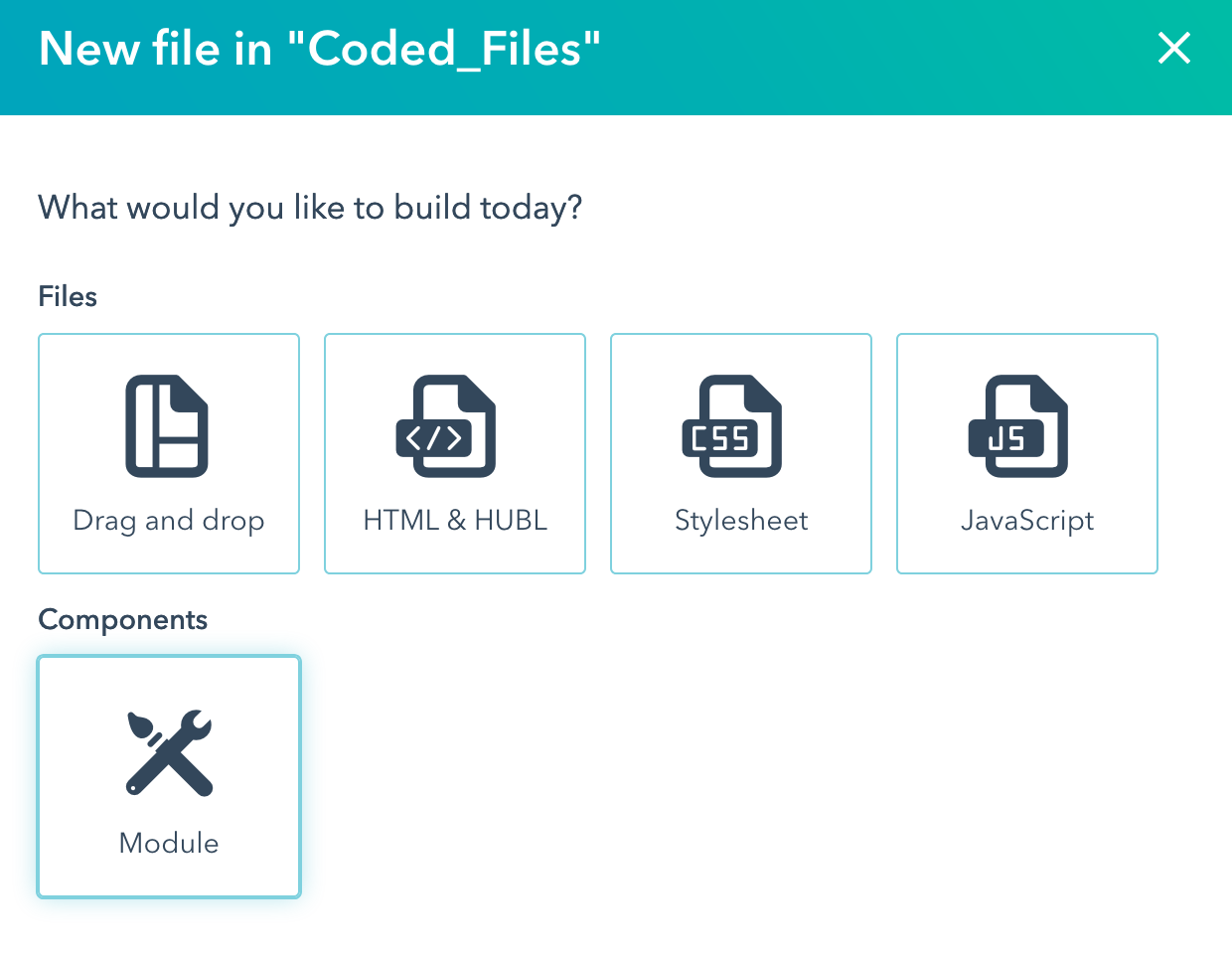The image consists of a user interface with a predominantly teal and white color scheme. 

At the top, there's a gradient teal box stretching from a more blue shade on the far left to a faint green on the far right. On the far left within this box, there's a white "X" symbol. Adjacent to it, bold white text reads: "New File in coded_files" with "coded_files" also in parentheses.

Beneath this teal box is a large white area followed by a black text prompt that asks, "What would you like to build today?" On the left side, the label "Files" is visible, under which there are four outlined boxes, each with a teal border and a white interior containing different icons and labels. 

From left to right:
1. The first box features an icon of a square with a folded upper right corner, beside a long line to the left and a short line at the bottom right. Below this icon, the label reads "Drag and drop".
2. The second box also has a square with a folded top right corner, showing a dark blue rectangular box with a white slash mark and two 'V' shapes facing opposite directions. The label underneath is "HTML & HUBL".
3. The third box mirrors the folded-corner square design with another dark blue rectangle, this time containing the letters "CSS" in white. Below it, the label says "Stylesheet".
4. The fourth and final box on the right showcases the same folded-corner design, dark blue rectangle with the letters "JS" in white, and is labeled "JavaScript".

Below the "Drag and drop" section, the term "Components" is highlighted. Furthermore, another box beneath "Components" is outlined with a blue border indicating selection. Inside this box, there's a wrench crossed with a narrow paintbrush forming an "X". The wrench stretches from the lower left to upper right, and the paintbrush extends from the bottom right to the upper left. Below this icon, the text reads "Module".